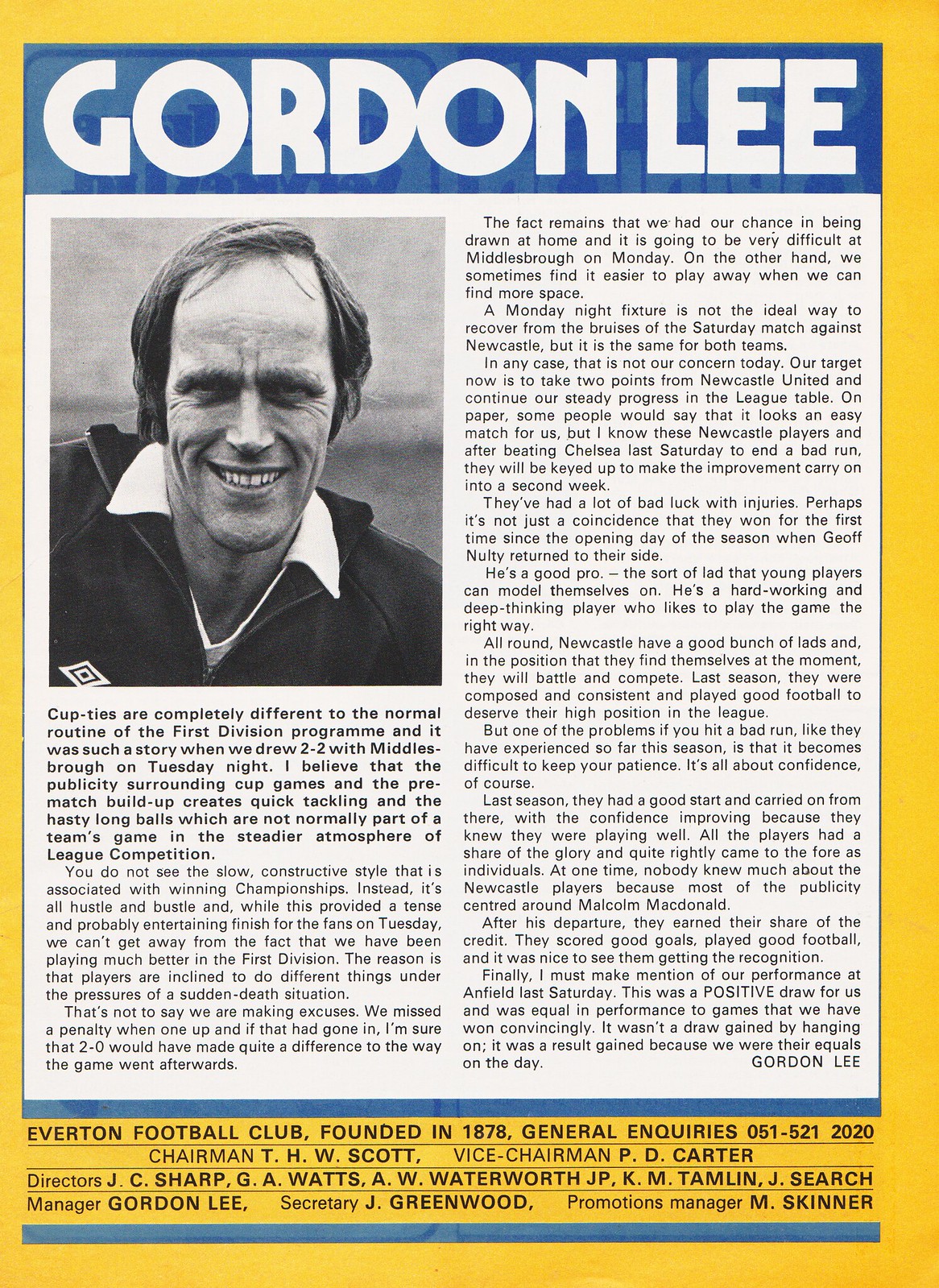The image features what appears to be an announcement handbill or the front cover of a sports magazine, likely related to a sporting event. Dominating the top of the page is a blue banner with "Gordon Lee" prominently displayed in white letters. A large portion of the upper section, approximately two-thirds, is dedicated to a photograph of Gordon Lee, the manager of Everton Football Club, intently looking ahead with a smile. A detailed two-column article accompanies the image, discussing the upcoming playoffs for Everton Football Club. The text delves into the challenges of an away game at Middlesborough following a tough match against Newcastle, touching on the difficulties of back-to-back fixtures. The bottom portion of the handbill, bordered by a gold frame, lists the club's officers, including the chairman, directors, promotion managers, and general inquiries phone number. The caption also highlights the club's founding year, 1878. The colors in the image, encompassing yellow, blue, white, black, and various shades of gray, give it a distinct and cohesive look, resembling a dedicated sports publication or program.